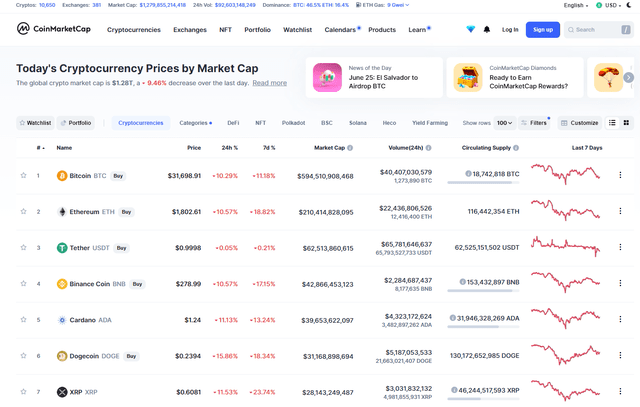The image predominantly features a white background with detailed content spread across various sections. At the top left corner, the website name "CoinMarketCap" is displayed in black text, accompanied by a small circular logo to its left. To the right of the website name, there are several navigation tabs with black text, including "Cryptocurrencies," "Exchanges," "NFT," "Portfolio," "Watchlist," "Calendars," "Products," and "Learn."

On the top right corner, there is a bright blue, rounded rectangular button with white text that reads "Sign Up." Next to it on the left is the black text "Log In."

The main body of the image consists of seven rows of information. On the bottom left side, there are light gray numbers stacked vertically from one to seven. Each number aligns with a corresponding row of black text paired with circular-looking symbols on the left side of the text.

On the bottom right side of each row, there are bright red graph lines indicating trends. These lines show varying movements but predominantly trend downwards across all rows. Additionally, there are three columns of gray text to the left of these red graph lines.

Overall, the image appears to be a structured layout of a website page from CoinMarketCap, featuring various navigational elements, user action buttons, and data rows indicative of cryptocurrency market trends.